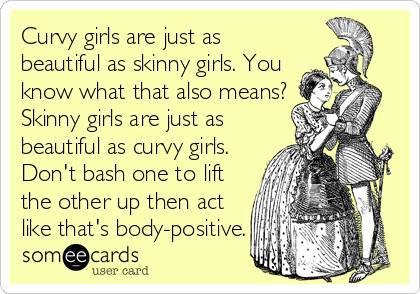In this image, we have a light, creamy yellow background featuring a meme with a motivational message. On the right side, there's a detailed, pencil-style illustration that seems reminiscent of Victorian art. The image depicts a man, possibly a French soldier with a large plume on his helmet and a sword on his hip, embracing a woman in a large, puffy dress. 

The focal point on the left side is a block of black text that reads: "Curvy girls are just as beautiful as skinny girls. You know what that also means? Skinny girls are just as beautiful as curvy girls. Don't bash one to lift the other up, then act like that's body positive."

The style of the overall graphic suggests that it is likely intended for social media sharing, with the purpose of promoting body positivity. The meme captures attention with its clear message against body shaming and the harmonious, albeit contrasting, illustration enhances its visual appeal. Created by SomeEEUserCard, this meme takes up the entirety of the image, presenting a unified and thought-provoking statement.